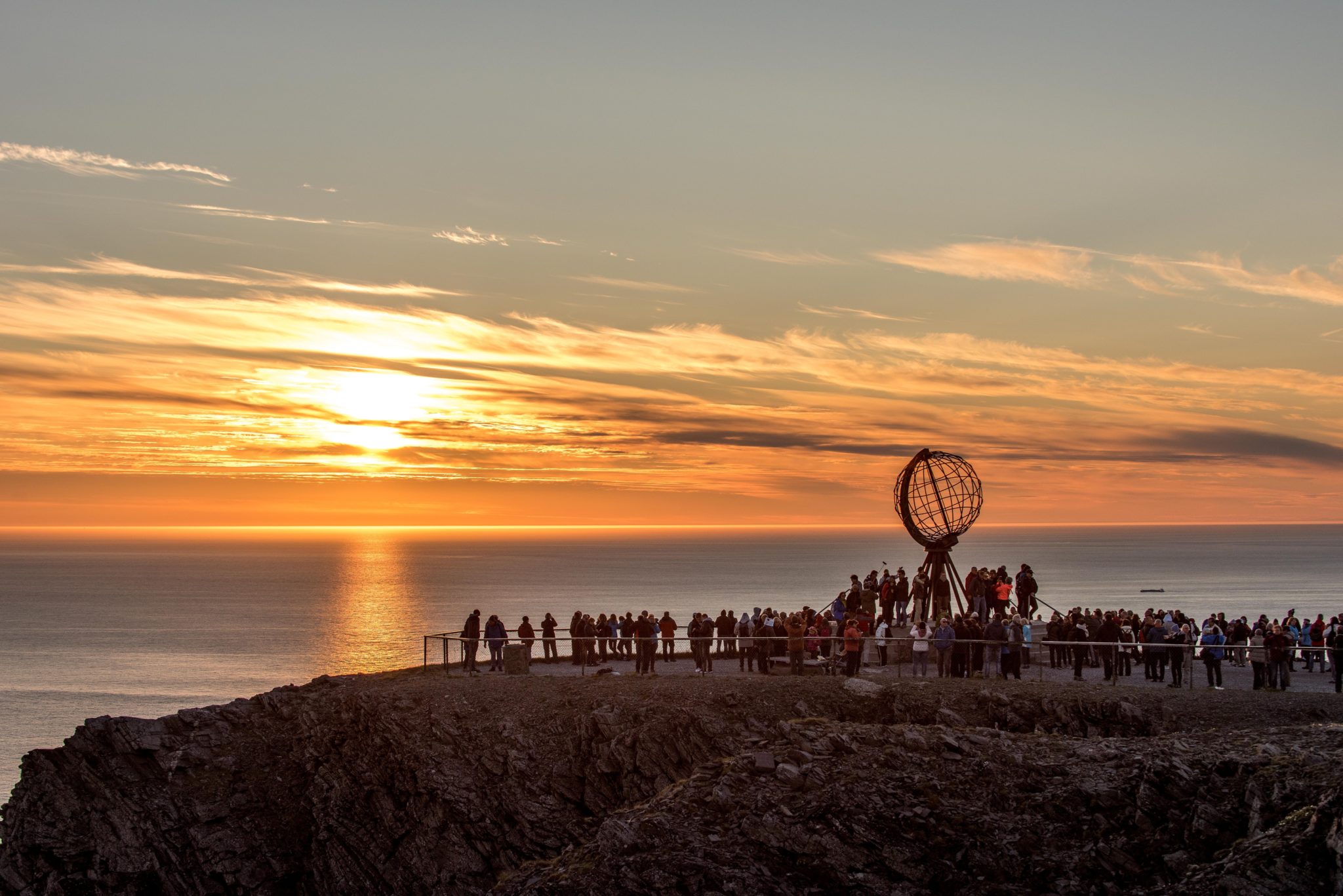The image captures a serene sunset over a calm ocean, with the sun low in the sky on the left, casting an orange-yellow glow and a conical reflection across the water. Partially cloudy skies frame the sun, adding texture to the horizon. In the bottom 20% of the image, a rocky cliff juts out, occupied by a large group of about 30 to 100 people, gathered near a guard rail. Among the onlookers, a prominent metal globe structure, about the height of two to three people, stands tilted at an angle in the center of the group. The area appears well-visited, with benches and a trash can nearby, enhancing the impression of it being a popular tourist spot.